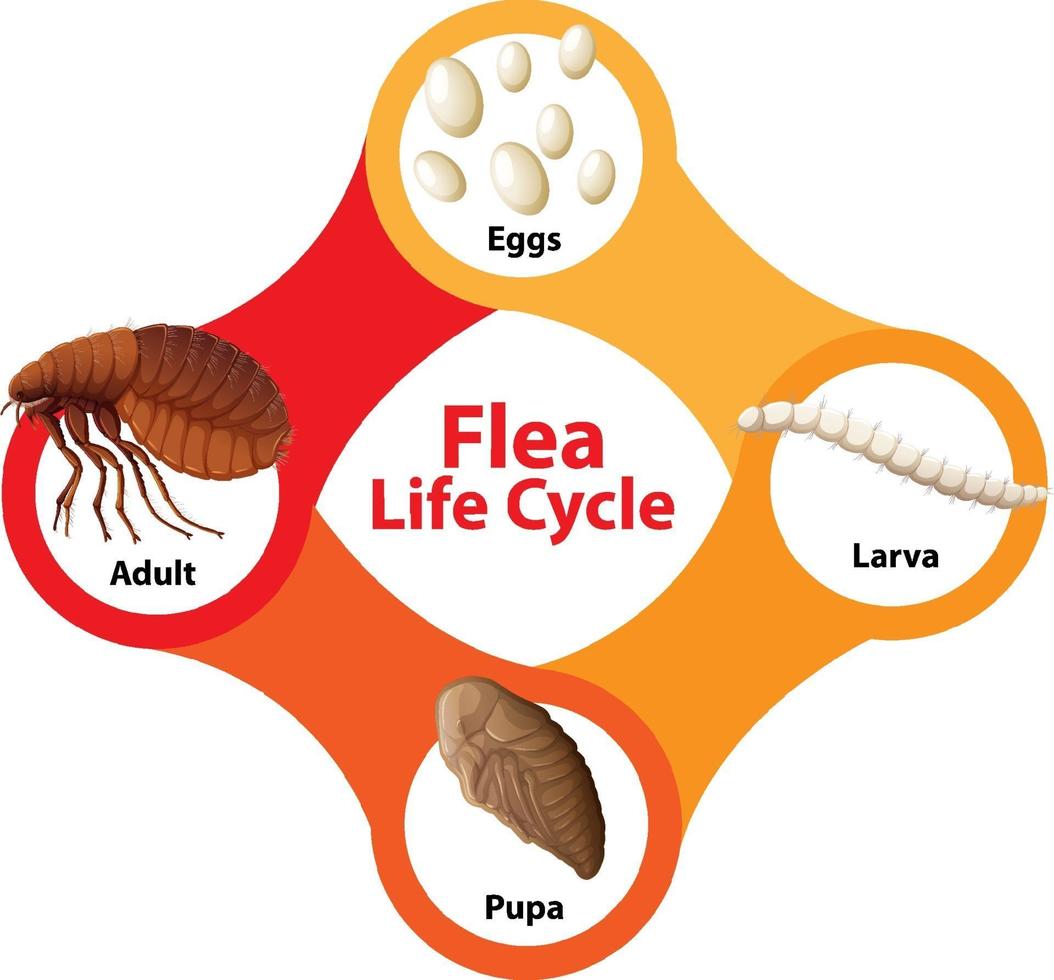The image is an educational and animated diagram with a white background that details the flea life cycle. At the center, in red text, it reads "Flea Life Cycle." The diagram is divided into four interconnected circles, each representing a stage in the life cycle, and connected by colored stripes in various shades of orange and red. 

At the very top, a light orange circle labeled "Eggs" in black text depicts off-white, oval-shaped eggs of different sizes. From there, an orange stripe leads to a darker orange circle on the bottom right labeled "Larva," showing a white worm-like larva. A subsequent orange stripe connects this to another, even darker orange circle in the bottom left labeled "Pupa," which depicts a bug encased in a cocoon-like form. Finally, a red stripe leads to the top left circle labeled "Adult," displaying a brown adult flea facing left. 

Black text descriptions accompany each stage: "Eggs," "Larva," "Pupa," and "Adult," guiding the viewer through the developmental stages of the flea. The primary colors used in the diagram are light orange, dark orange, red, and white, effectively illustrating the transformation from egg to adult flea.